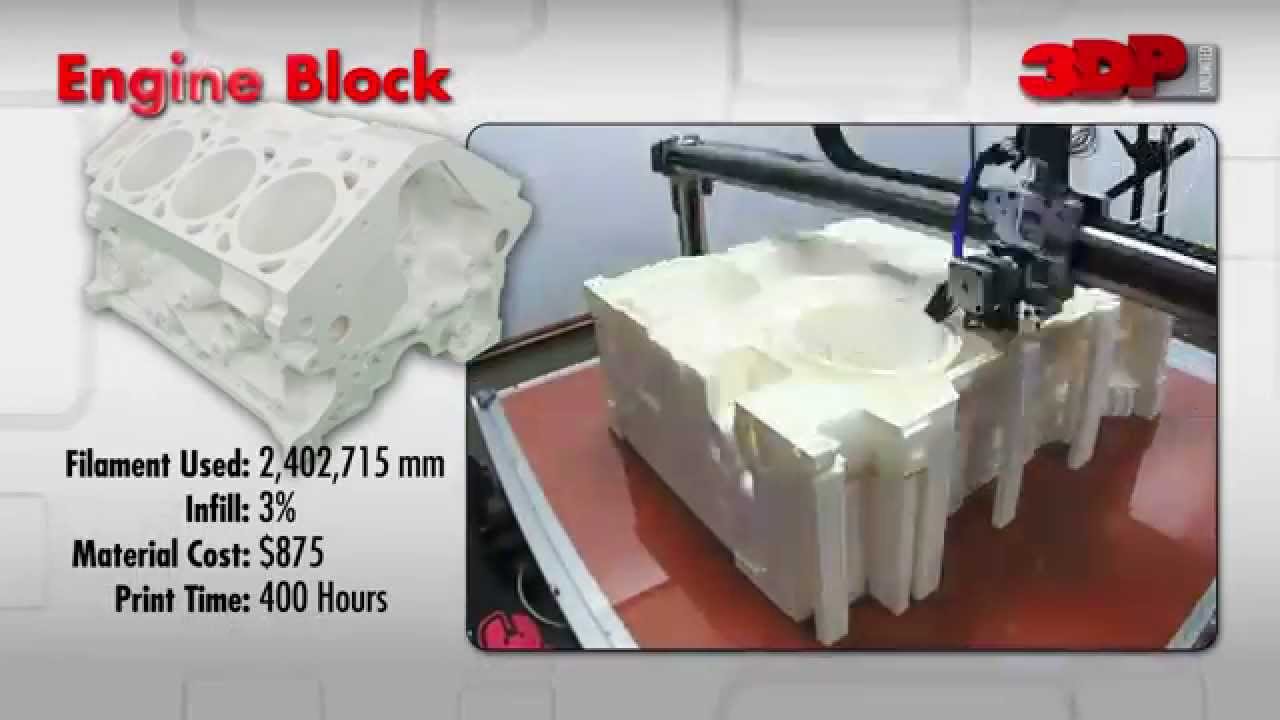The image features a grey background with the focal point being a detailed 3D printing process. Dominating the right side is a photograph of a sophisticated 3D printer actively printing a white engine block, which is approximately halfway complete. The top right corner displays "3DP" in bold red font, affirming the 3D printing technology. In the top left corner, the words "engine block" are prominently featured in red letters. Below this text is a smaller image showcasing a white 3D model of the engine block. To the left of the main 3D printer photograph, black text provides specific details about the printing process: "Filament used: 2,402,715 millimeters; Infill: 3%; Material cost: $875; Print time: 400 hours." The overall aesthetic is clean and technical, highlighting the intricate and costly nature of 3D printing technology used for manufacturing engine blocks.